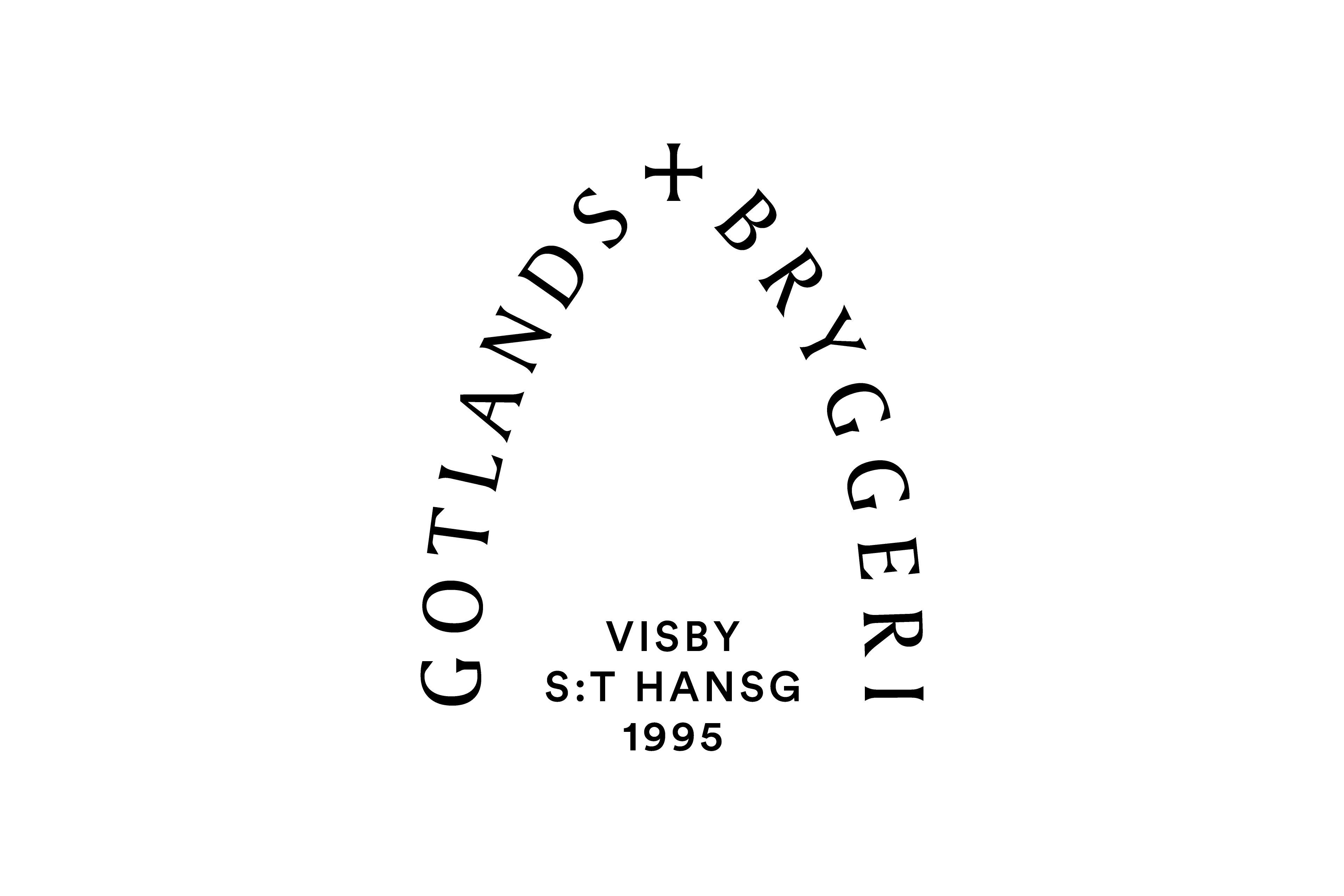The image features a logo with black text arranged in a conical shape on a white background, creating the illusion of the text floating in a white void. The logo appears to be for a company or manufacturer, possibly a brewery, as suggested by the repeated mention of words like "Gotlands" and "Bryggeri." At the top of the conical text arrangement, there is a cross, indicating a possible association with tradition or heritage. The text reads "GOTLANDS BRYGGERI VISBY S:T HANS G 1995," suggesting it is not in English but seems to spell out "Gotlands Bryggeri Visby S.T. Hans G, 1995." The centered, minimalist design and the combination of black text on a white background make for a clean and striking visual. This logo could be used on various mediums, such as signage, websites, or merchandise like T-shirts.